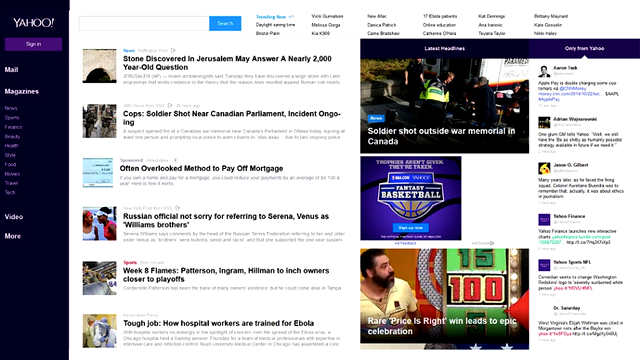A detailed screenshot of the classic Yahoo home page is depicted. At the top left, the recognizable Yahoo logo stands prominently above a purple button with white text prompting users to sign in. Adjacent to it, a menu bar is available, containing options for "Mail" and "Magazines," followed by a comprehensive list of links, although the entirety of the list isn't legible. Clearly visible options include "News," "Sports," "Finance," "Beauty," "Health," "Style," "Food," "Movies," and "Travel," among others that are not discernible.

Below the menu bar, a series of sections is present. The first is dedicated to videos, succeeded by another labeled "More." On the far right, a search bar is for user convenience, beneath which several trending topics and various news articles from different media sources are displayed. Prominent stories include "Stone Discovered in Jerusalem May Answer a Nearly 2,000-year-old Question" and "Cop Soldier Shot Near Canadian Parliament: Incident Ongoing."

To the right of the news articles, a section filled with diverse advertisements and noteworthy video clips is visible. Adjacent to this is the "Only from Yahoo" segment, resembling social media updates with posts from varied accounts, complete with avatars. Some posts are from official Yahoo accounts such as Yahoo Finance and Yahoo Sports NFL. The page radiates an old-style Yahoo aesthetic, characterized by its distinct white and purple color scheme.